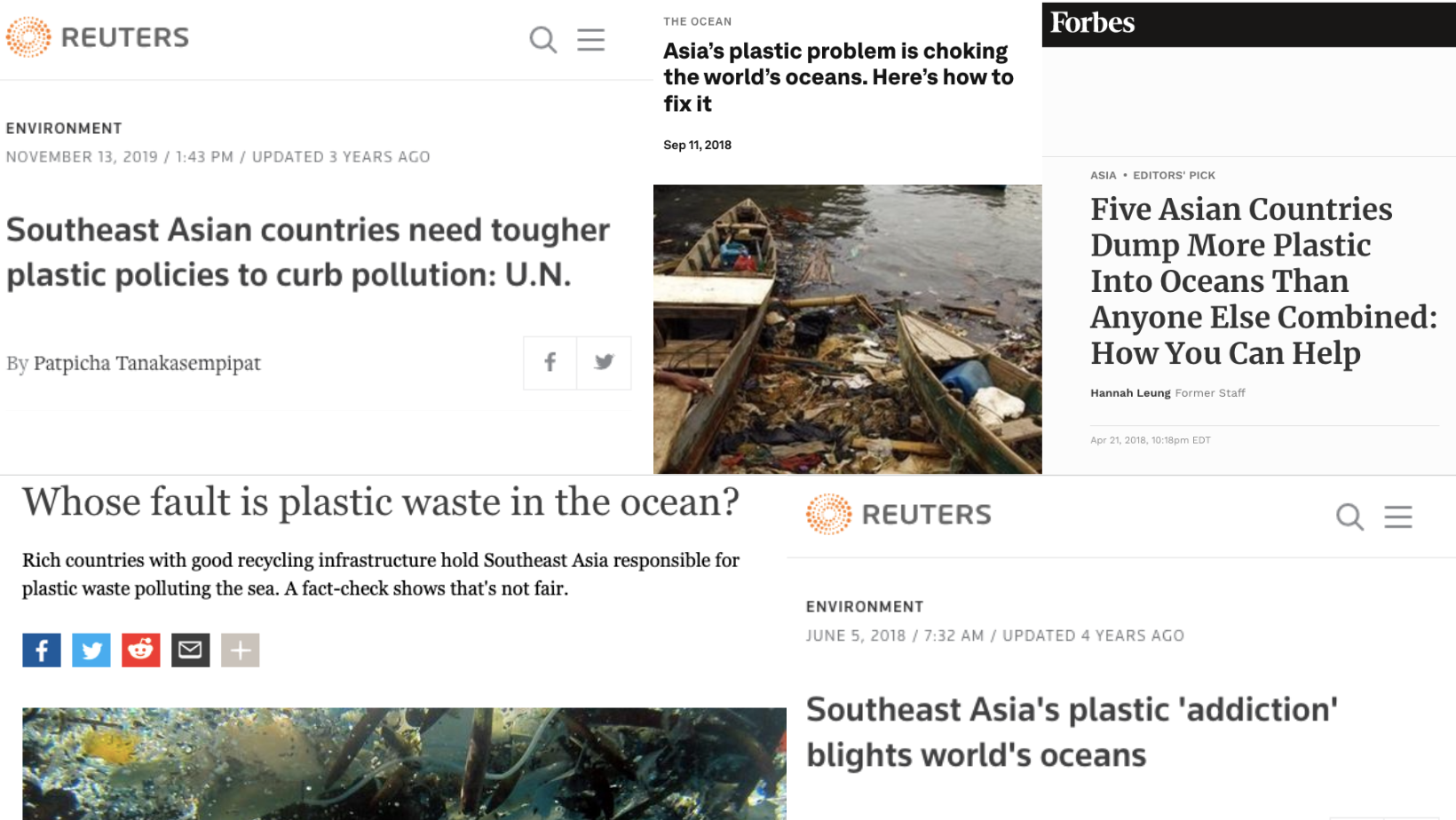**Detailed Caption:**

The screenshot features an article with a white background from Reuters, recognizable by the logo. The interface includes a magnifying glass icon, indicating a search function, and a hamburger icon, suggesting a menu option. The heading reads: "Southeast Asian countries need tougher plastic policies to curb pollution." The article is dated November 13, 2019, at 1:43 p.m., and was updated three years ago. Another segment highlights contributions from U.N. official Bipachanthanasem Pipat, emphasizing the dire plastic problem in Asian oceans and potential solutions.

Additionally, there is a section dated September 11, 2018, from Forbes, with the title “Five Asian countries dump more plastic into the ocean than anyone else. How can you help?” This part is marked by the recognizable Forbes logo, white text on a black rectangle, and categorized under “Asia” and “Editor's Pick.” Another snippet is from the environment section dated June 5, 2018 at 7:32 a.m. The combined content addresses the critical issue of plastic pollution in Asian oceans and seeks to identify accountability and suggest corrective measures.